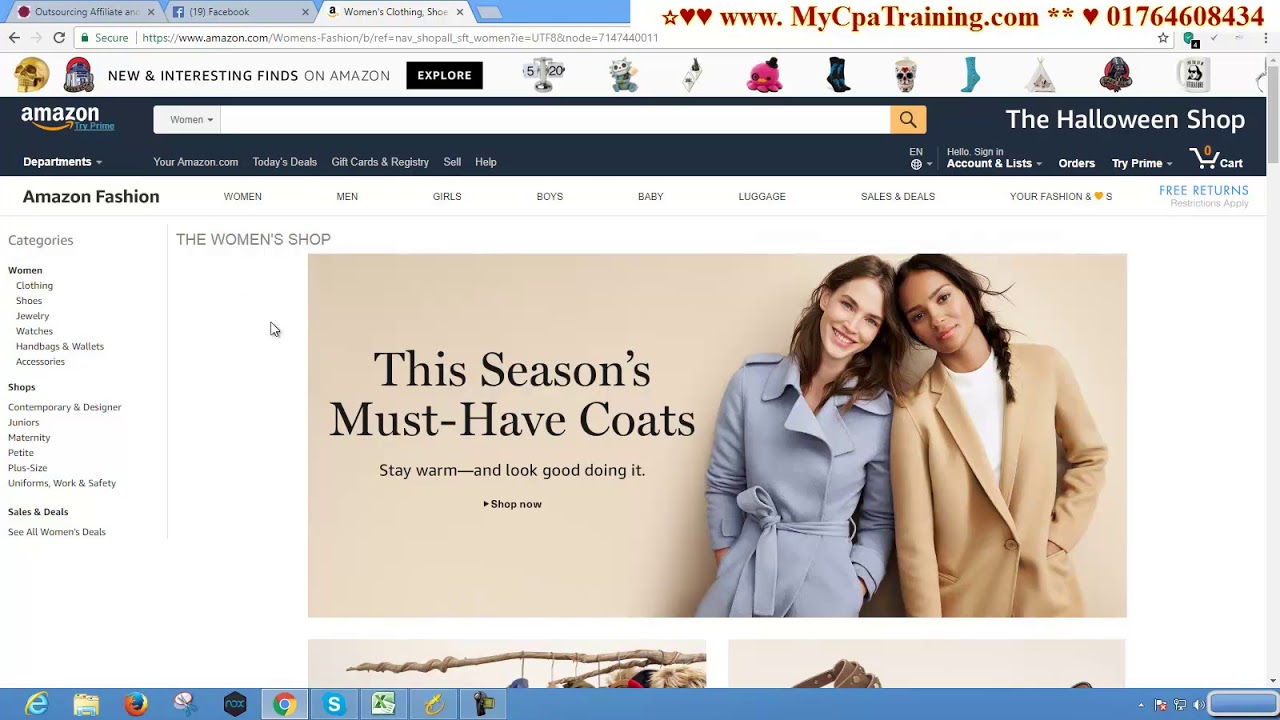This is a web page description for an Amazon shopping session, detailing the full layout and elements visible in the browser window.

---

On this Amazon webpage, the current URL reads "amazon.com/womens-fashion," indicating the user is browsing women's fashion. The browser shows two additional tabs: one with a Facebook symbol labeled "19 (Facebook)," and the other displaying what appears to be a red octagon with the text "outsourced and affiliate."

At the top-right corner of the screen, another URL is visible: "www.mycpatrainer.com," highlighted in red and accompanied by two stars and a heart symbol, alongside a red string of numbers: "017646084834."

On the Amazon page, a blue border spans the top with the word "Amazon" on the left, accompanied by the signature orange arrow icon. To the right of this icon, "Try Prime" is written in blue. A prominent white search bar, rectangular in shape, runs across the top of the page, transitioning to an orange section with a black magnifying glass icon at its far end.

The user is currently navigating the "Women's" tab. Adjacent to it, there is a link to the "Halloween Shop." Several main navigation tabs are displayed, including "Departments," "Amazon.com," "Today's Deals," "Gift Cards & Registry," "Sell," and "Help." Further right, personal account options appear: an "E" icon, "Hello, Sign-In," "Accounts," "Orders," "Try Prime," and a shopping cart icon with a "0" indicating no items in the cart.

Dominating the central area is an image featuring two models wearing jackets—one gray and one beige—set against a beige background. The black text next to the models reads, "This season's must-have coats. Stay warm and look good doing it," followed by a "Shop now" call-to-action.